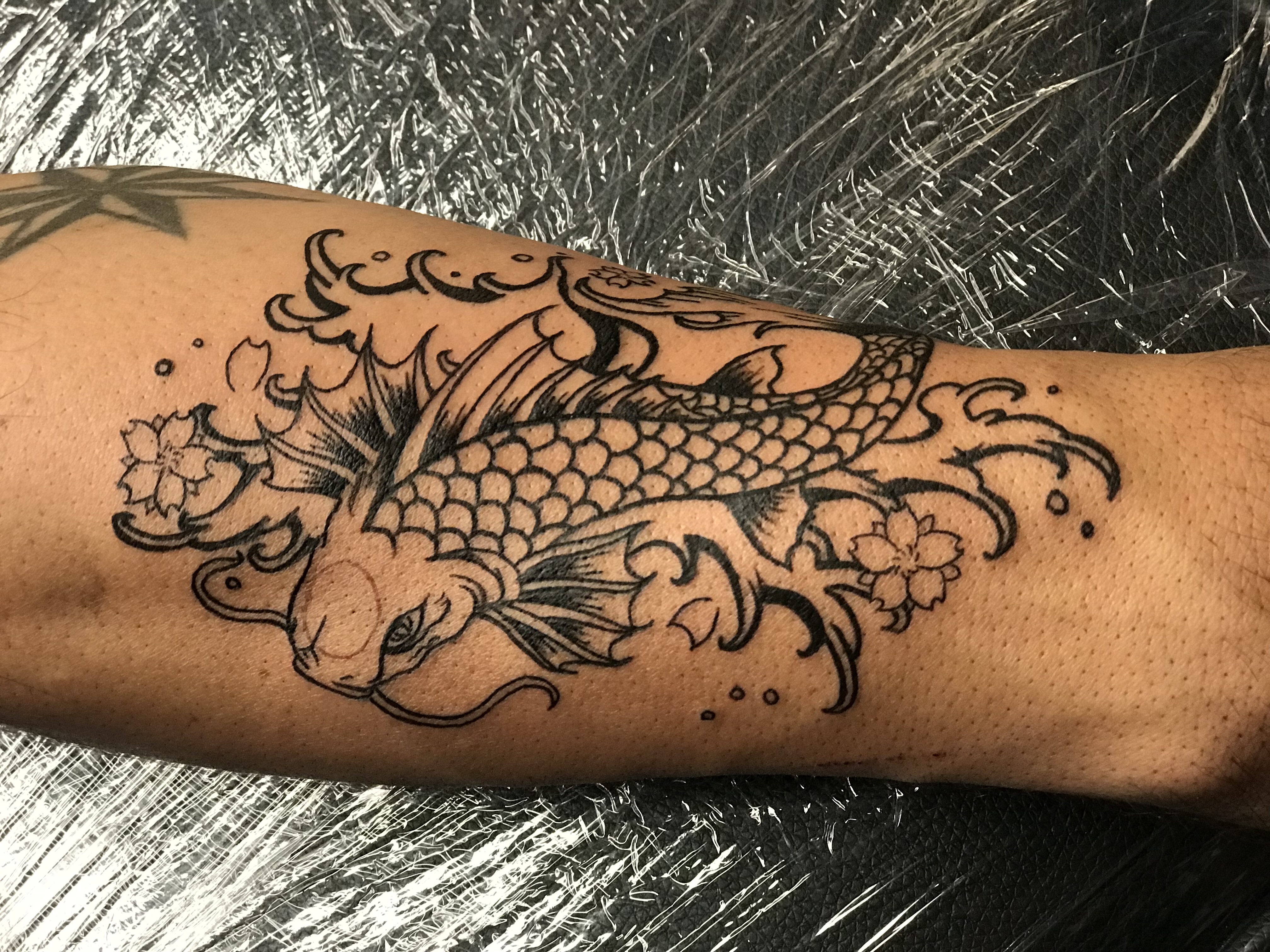This photograph captures a freshly-inked, black-and-white tattoo on a person's forearm, which is resting on a table covered in clear plastic wrap. The tattoo, positioned diagonally from the upper left down to the right, features an intricately detailed koi fish facing downward. The fish has visible whiskers, a prominently shaded fin, and scales across its body. Surrounding the koi are artistic depictions of flowers, petals, and splashing water, creating a dynamic and fluid design. Details include waves both above and below the fish, and three small circles below it. Additionally, there is a faded star tattoo near the upper left of the forearm. The entire scene is set against a background of shiny, wrinkled plastic wrap, emphasizing the freshness of the tattoo.